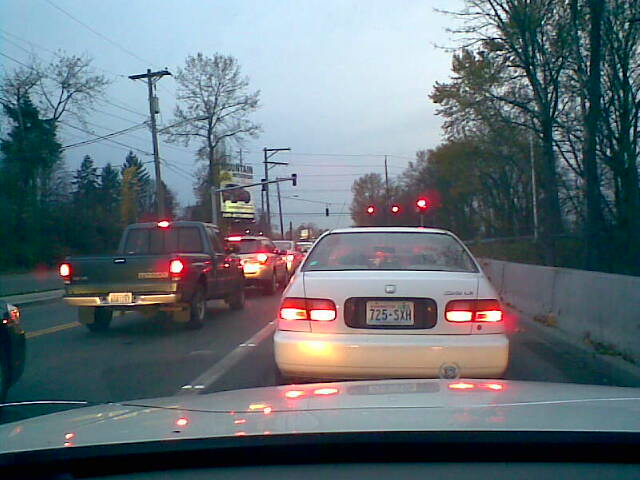The photograph is a detailed color snapshot taken from the driver's seat of a car, capturing the scene through the windshield. It depicts a typical traffic scenario on what appears to be either a dark, rainy day or the brink of nighttime. Directly in front of the viewer is a car with Washington state license plates, its taillights glowing a vivid red. The driver seems to be positioned in the right-hand lane, with a cement barrier lining the right side of the road. Beyond this barrier, a line of trees stretches into the distance. To the left, there is a green truck slightly ahead, surrounded by a series of cars both in front and behind it. In the distance, various telephone poles and additional trees are visible, along with a couple of traffic lights that hint at the controlled intersections further along the way. The overall atmosphere suggests a cautious journey through an urban environment under subdued lighting conditions.